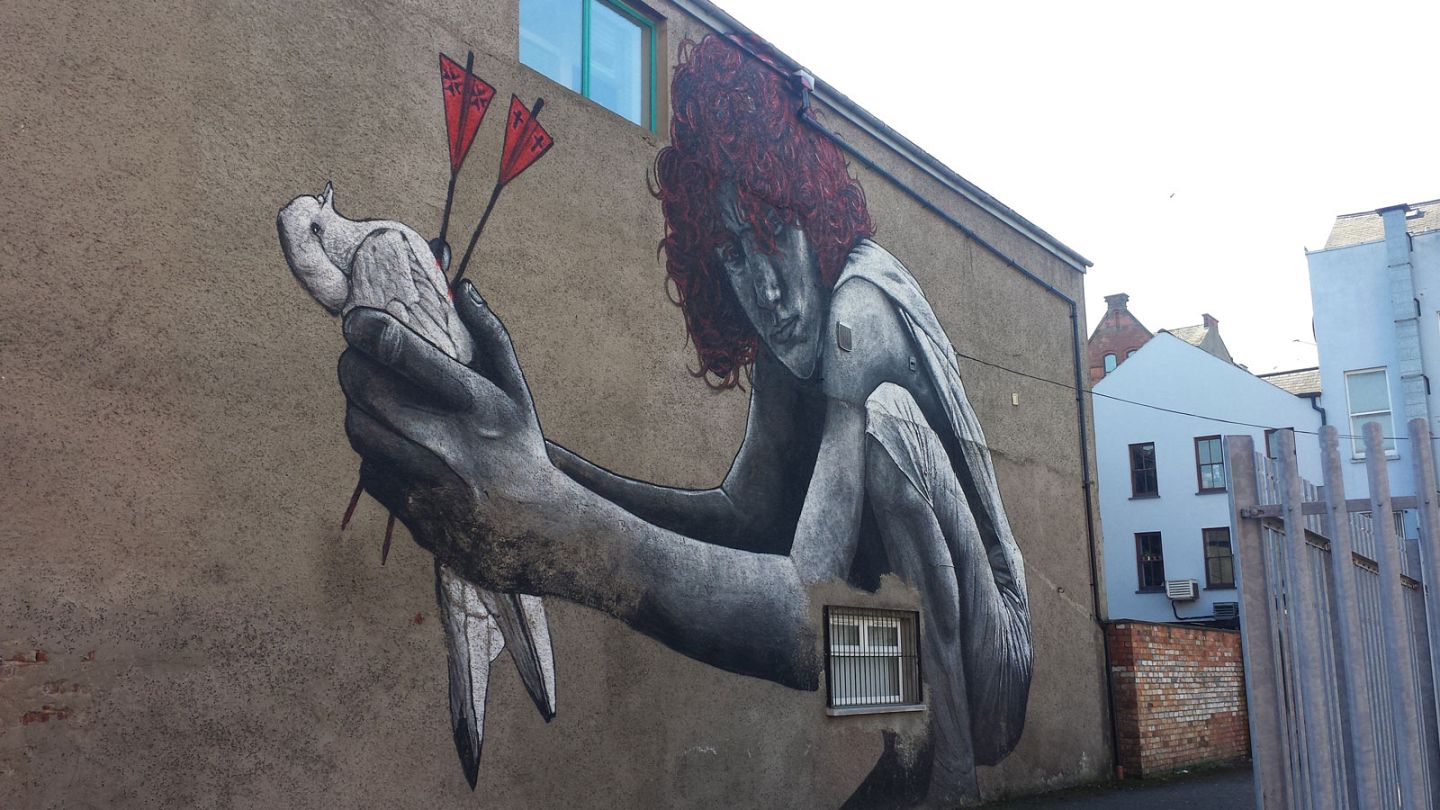This horizontally rectangular full-color photograph captures an outdoor scene under natural light. Dominating the image is a tan, brown stucco-style, two-story building featuring a striking mural on its side. The mural depicts a red-haired figure, who could be perceived as either a boy or a woman, crouching and holding a white bird—either a pigeon or a dove—pierced by two red arrows in the heart and showcasing red tail feathers. The bird appears lifeless, its head resting backward. The person's clothing is predominantly gray and somewhat indistinct. The mural is central, with a window featuring blue-tinted glass visible to the left of the figure's head.

Surrounding the central building, a white sky occupies much of the upper right corner, indicating clear weather. Additional architectural elements provide context: to the right of the mural, white buildings appear in the background, along with a red brick wall and a brown wooden fence panel at the bottom right. A sliver of ground is visible, but the mural remains the primary focus.